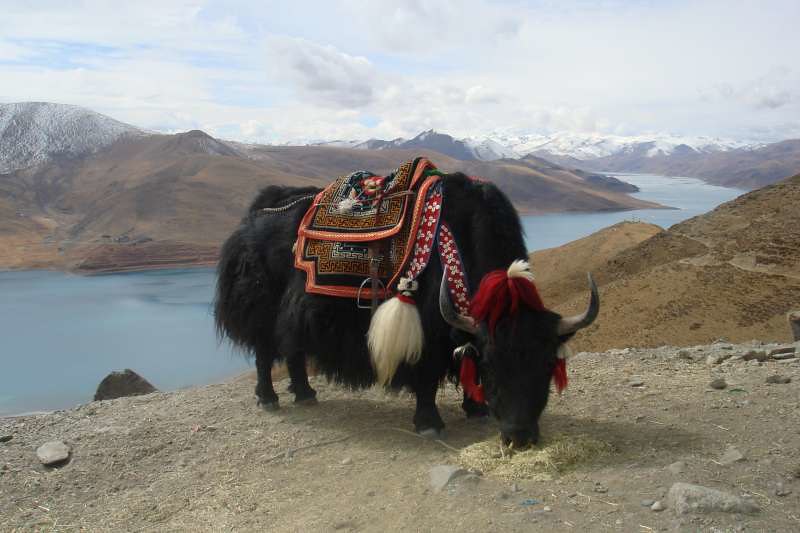The photograph depicts a large, shaggy black bull with curved black and gray horns, leaning down to eat hay or straw from a pile on a patch of bare ground dotted with rocks. The bull is adorned with an ornate saddle featuring a vibrant orange, black, and red geometric pattern, along with a visible stirrup hanging from a leather strap. Additionally, the bull wears a maroon and white headgear, which includes a strap ending in a white tassel. Surrounding the foreground are mountainous landscapes with a river winding between the dark brown terrain. The most distant mountains are capped with snow and fluffy clouds drift in the sky above.